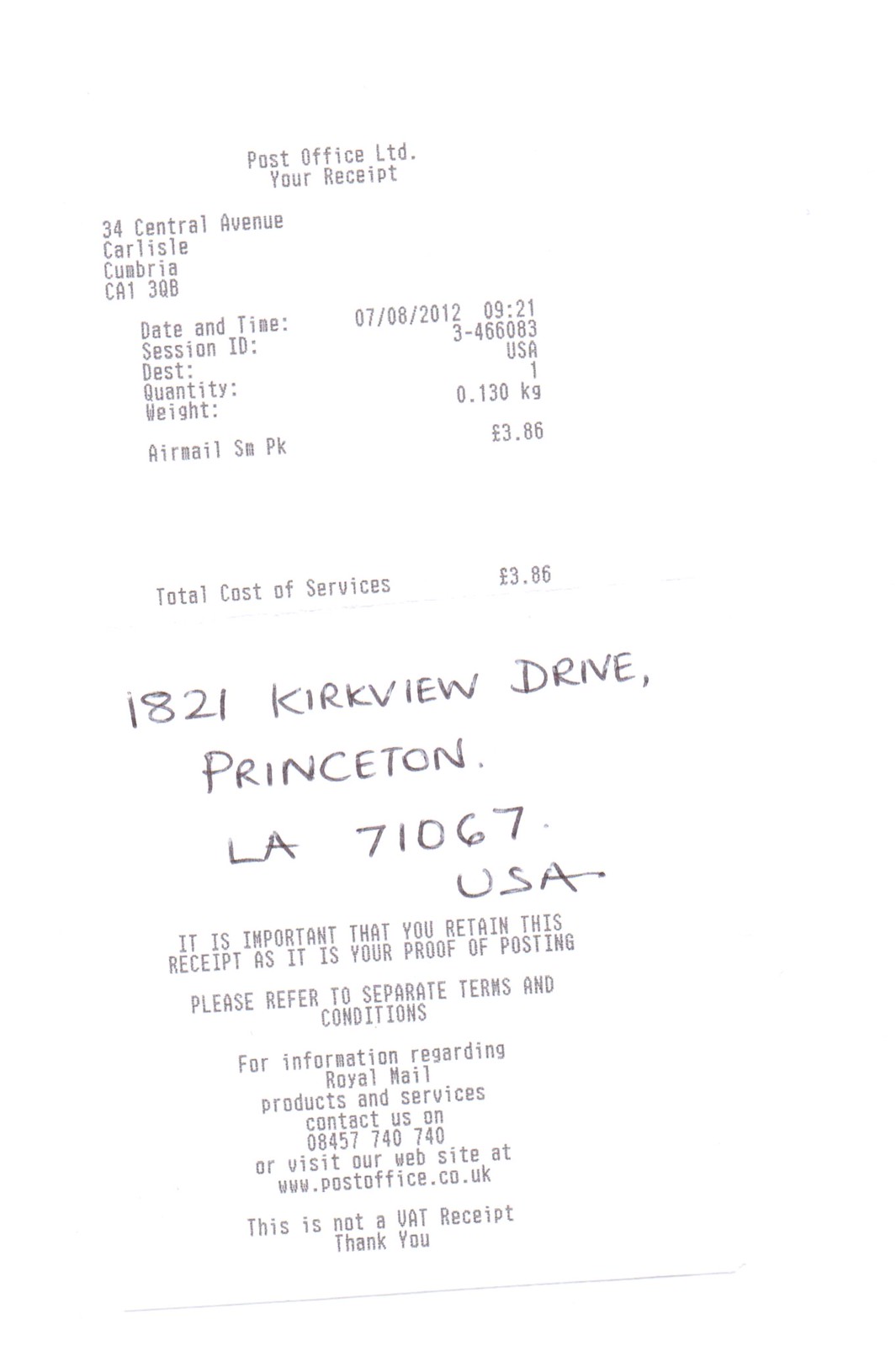**Detailed Caption:**

This image showcases a receipt from the Post Office Ltd., situated at 34 Central Ave, Carlisle, Cumbria, CA1 3Q8. The receipt confirms the provision of postal services and lists essential transaction details such as the date, time, session ID, destination, quantity, weight, the type of mail (air mail), and the classification of the parcel (small package). The total cost of the services rendered amounts to £3.86. Notably, the middle section of the receipt features a handwritten address: 1821 Kirkview Drive, Princeton, LA 71067, USA. At the bottom of the receipt, there is a note emphasizing the importance of retaining the receipt as proof of posting. This section also suggests consulting separate terms and conditions for further information on Royal Mail products and services, provides a contact number and website, and clarifies that this document is not a VAT receipt. The text concludes with a courteous "Thank you."